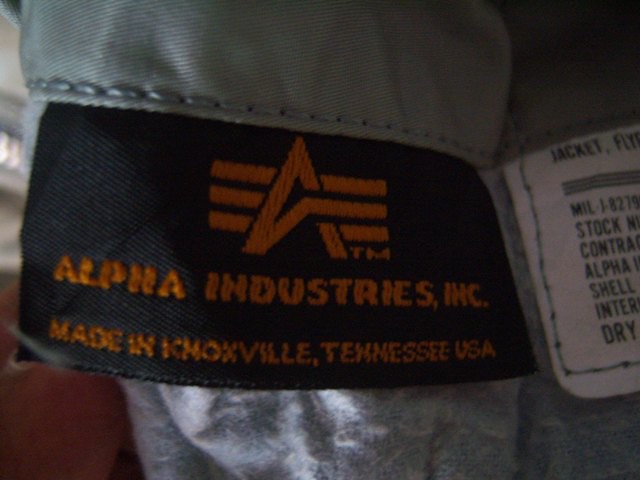The image depicts a piece of clothing turned inside out, revealing a black rectangular tag. The tag features an orange symbol consisting of the letter "A" flanked by lines, and the trademark "TM." Below the symbol, the text "Alpha Industries Inc." is displayed in the same vibrant orange color. The tag indicates that the garment was made in Knoxville, Tennessee, USA. Surrounding the black tag are details of the inside of the garment, suggesting it is likely a jacket. Adjacent to the black tag is a white tag with a considerable amount of black text and a small red mark in the lower left-hand corner. The white tag appears to provide additional information about the jacket, potentially describing its filling and other specifications. The contrasting tags and the visible seam details confirm the garment's inside-out orientation.